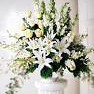This image is a thumbnail-sized, low-resolution studio shot of a bouquet of flowers, making it very pixelated and somewhat difficult to distinguish details. Despite this, it can be discerned that the bouquet is predominantly composed of white flowers, possibly including lilies and carnations, interspersed with pale yellow or light green hues. The arrangement sits atop a white pedestal or a small column-like structure, contrasting against a very white, presumably studio curtain background. The bouquet is lush with green leaves, though the dark green foliage is somewhat indistinct. The composition fills most of the frame, focusing on the intricate interplay of white blooms and greenery.